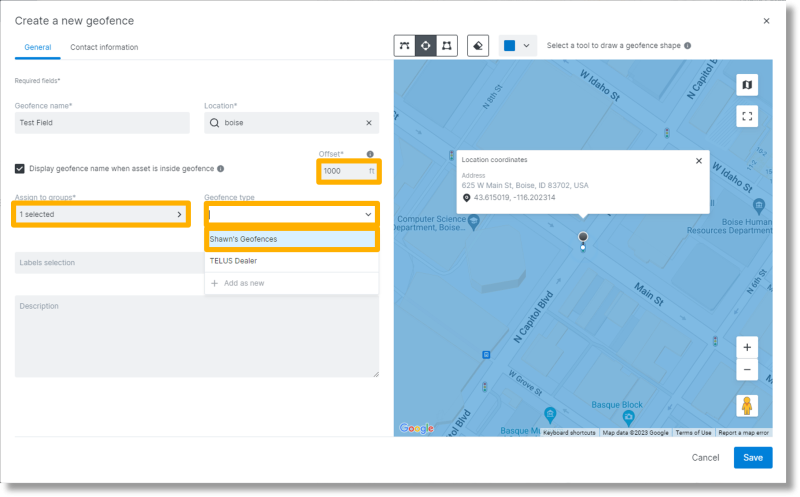**Detailed Caption:**

The screenshot displays a webpage from a geofencing application with the heading "Create a New Geofence". At the top of the page, there are several control buttons and symbols, including a general button and a contact information button. The interface is replete with buttons, drop-down menus, and various interactive elements.

Enlarging the image reveals that this geofence is named "Sean's Geofence". Inside the "Geofence Name" text box, we see "Test Field". The geofence's location is specified as Boise, Idaho. There's an option selected to display the geofence name when an asset is inside the geofence. The offset distance is set to 1,000 feet. Only one group has been assigned to this geofence as indicated under "Assign to Groups".

Further details include a drop-down menu for "Geofence Type". The label selection for this geofence includes "TELUS Dealer". Beneath these settings is a description box.

On the right side of the page, there is a map displaying the geofence's precise location. The address listed is 625 West Main Street, Boise, Idaho, 83702, USA. The coordinates provided are latitude 43.615019 and longitude -116.202314, pinpointing the exact intersection of North Capitol Boulevard and Main Street.

The heading "Create a New Geofence" is prominently displayed, accompanied by various selections and drop-down menus to complete the setup of Sean's Geofence in Boise, Idaho.